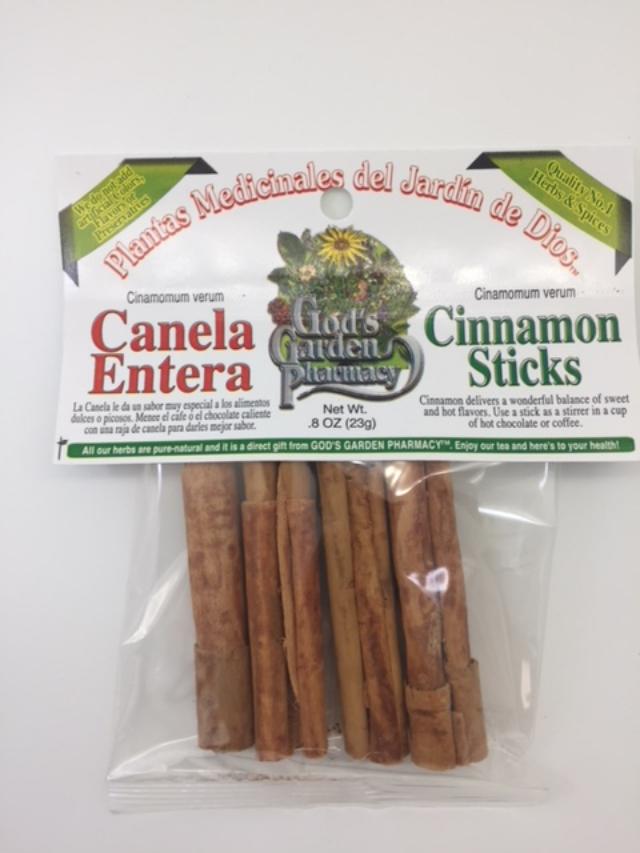The image depicts a package of cinnamon sticks. The top portion of the packaging is made of paper, while the bottom part is a clear plastic bag showcasing four cinnamon sticks. The center of the package features a prominent logo with a colorful illustration of a small garden containing sunflowers and various other flowers. Superimposed on this floral background is the text "God's Garden Pharmacy." Surrounding the logo, the text reads “Plantes Medicinales del Jardin de Dios” in Spanish, and includes bilingual descriptions such as “Cinnamom Verum,” “Canela Entera,” and “Cinnamon Sticks.” The package also highlights selling points in English, stating “Quality Number One,” “Herbs and Spices,” and provides instructions on how to use the cinnamon sticks for hot chocolate or coffee. The net weight is marked as 8 ounces. The overall aesthetic of the packaging is both informative and visually appealing, with elegant detailing in the floral design.